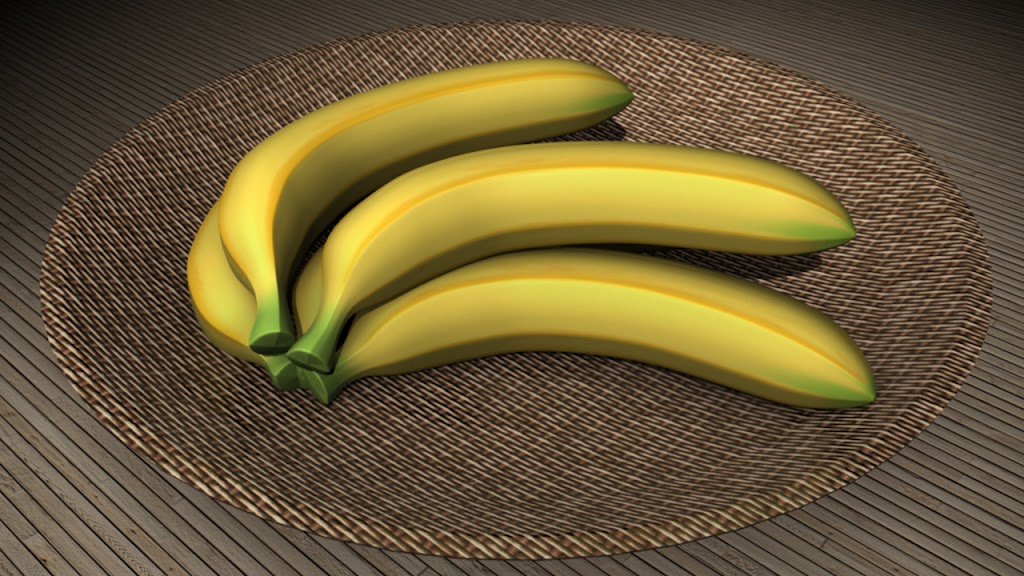The image depicts a well-lit, horizontally oriented 3D-rendered scene featuring a bundle of five bananas laid atop a shallow, intricately woven wicker bowl. Three bananas are prominently visible, with their yellow bodies and distinctive green tips indicating their freshness, while the other two bananas are partially hidden beneath them. The woven bowl, which exhibits a detailed brownish-white pattern, rests on a surface of wooden slats in varying shades of brown and gray. The background gradually fades into darker shadows in the top left and top right corners, further enhancing the realism and depth of the scene. This meticulously designed image lacks any text, reinforcing its appearance as a professional, computer-generated illustration rather than a traditional photograph.